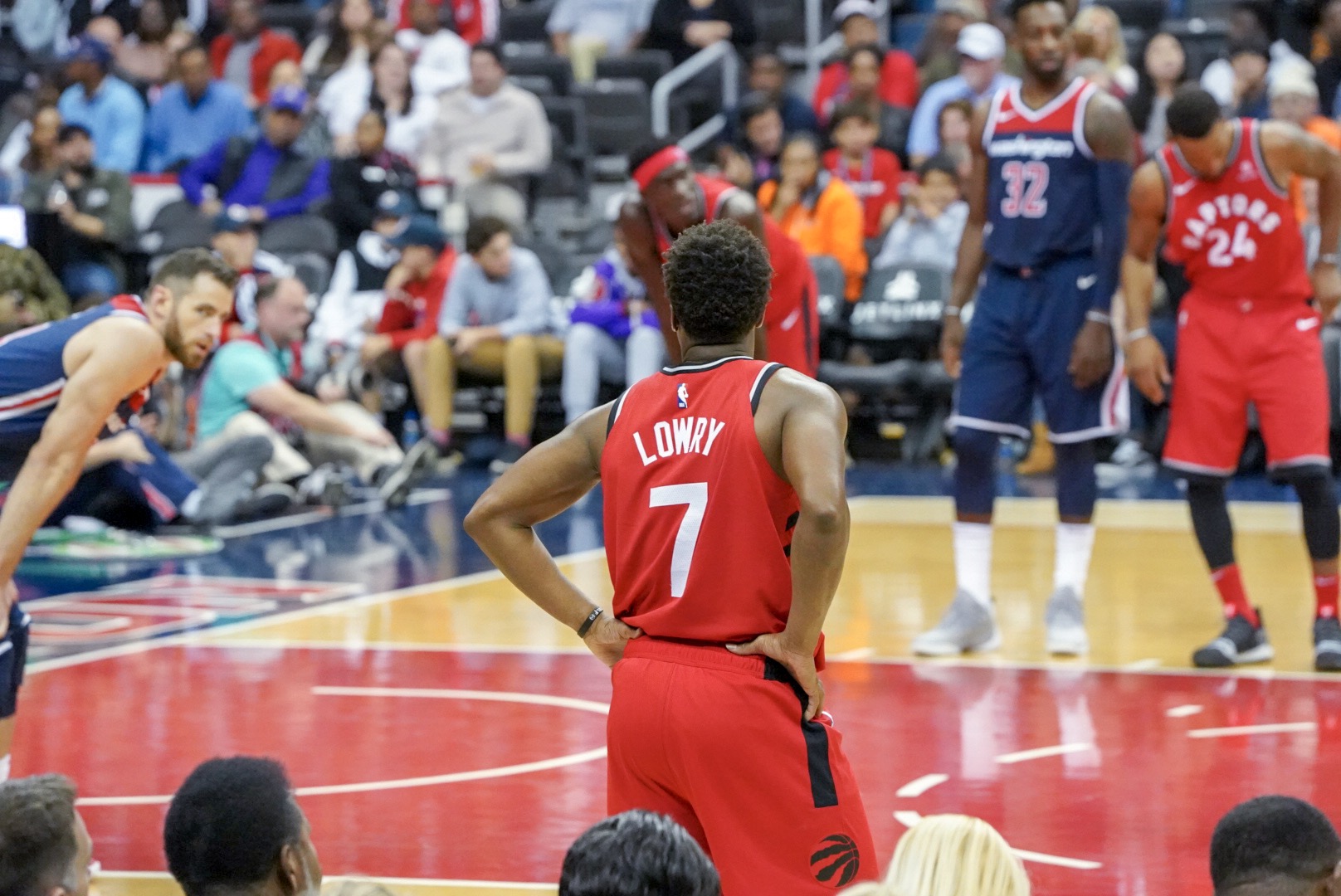This horizontal rectangular image captures an intense moment during a basketball game. The photograph, taken from within the crowd, includes the backs of spectators' heads at the bottom of the frame. In the background, we see about three or four rows of fans in the stands, suggesting a full stadium.

The focal point of the image is at the foul line, where players from both teams are positioned. The court is visually striking with its dark blue boundary and a red-painted key area marked by white circles. 

At the center, a black player in a red jersey with white text "Lowry 7" stands with his hands on his hips, seemingly ready to assert himself. To the left, a white player in a blue, white, and red jersey is bent over with his hands on his knees. On the right side of the frame, two men stand close to each other; one in a blue, red, and white jersey, and a black man in a red and white jersey displaying "Raptors 24" on the front. The presence of the players and the described context suggest that the game may be paused for a free throw.